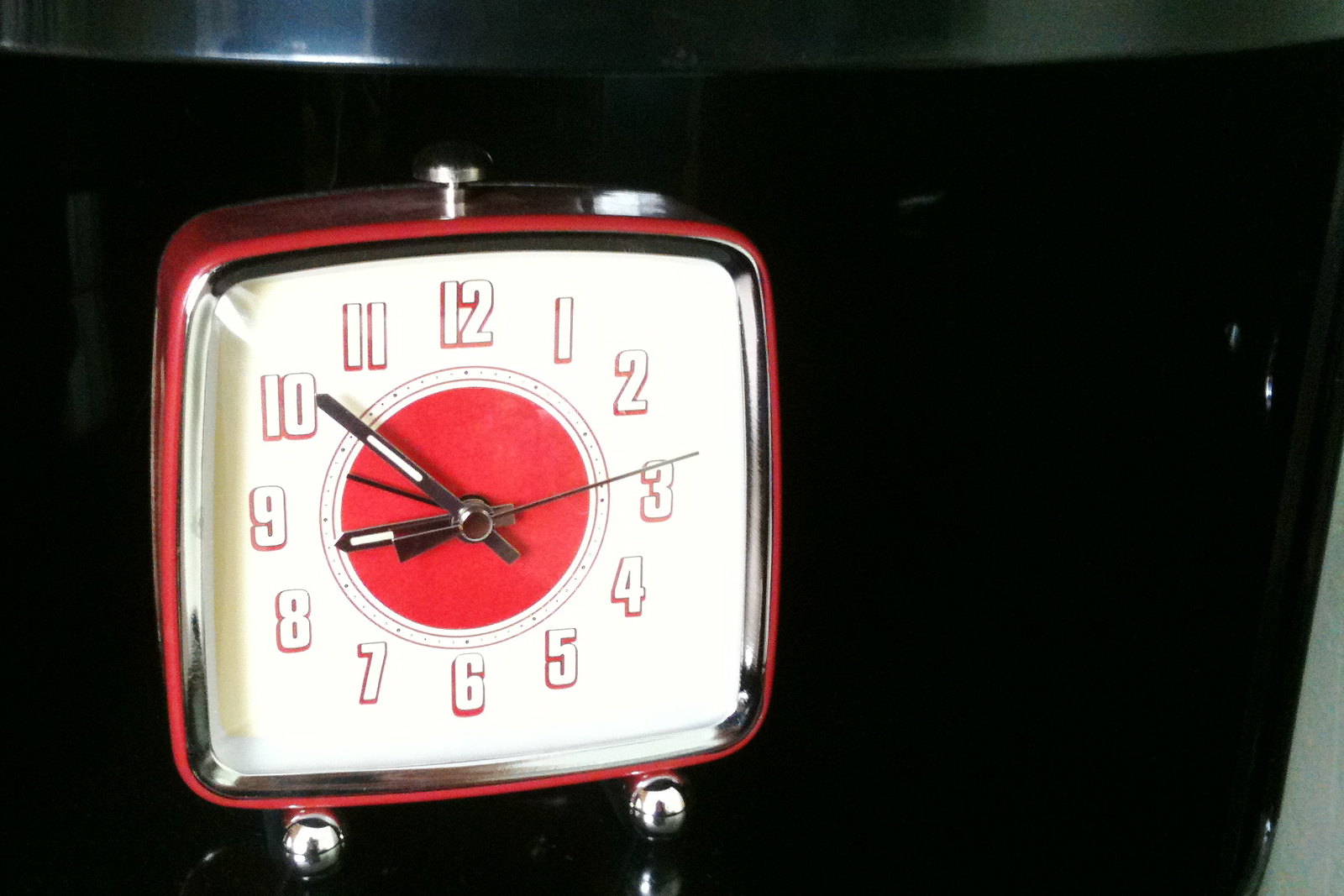The image is a detailed color photograph of a retro-style alarm clock set against a predominantly black background with subtle gray and olive-green hints on the edges. The clock itself has a square shape with softly rounded corners and a striking red metal frame. The clock face is cream-colored and features large black hands with white filling, situated on a red circle at the center. This red circle is outlined by thin red rings. The large numbers around the clock face are white and meticulously trimmed in red. At the top of the clock, there is a silver screw-like button, likely for turning off the alarm. The clock stands on two silver bead-like feet. The photograph background highlights the clock, making the vibrant details more pronounced, with a metallic outline visible in the upper left and a dark olive-green section in the bottom right corner.